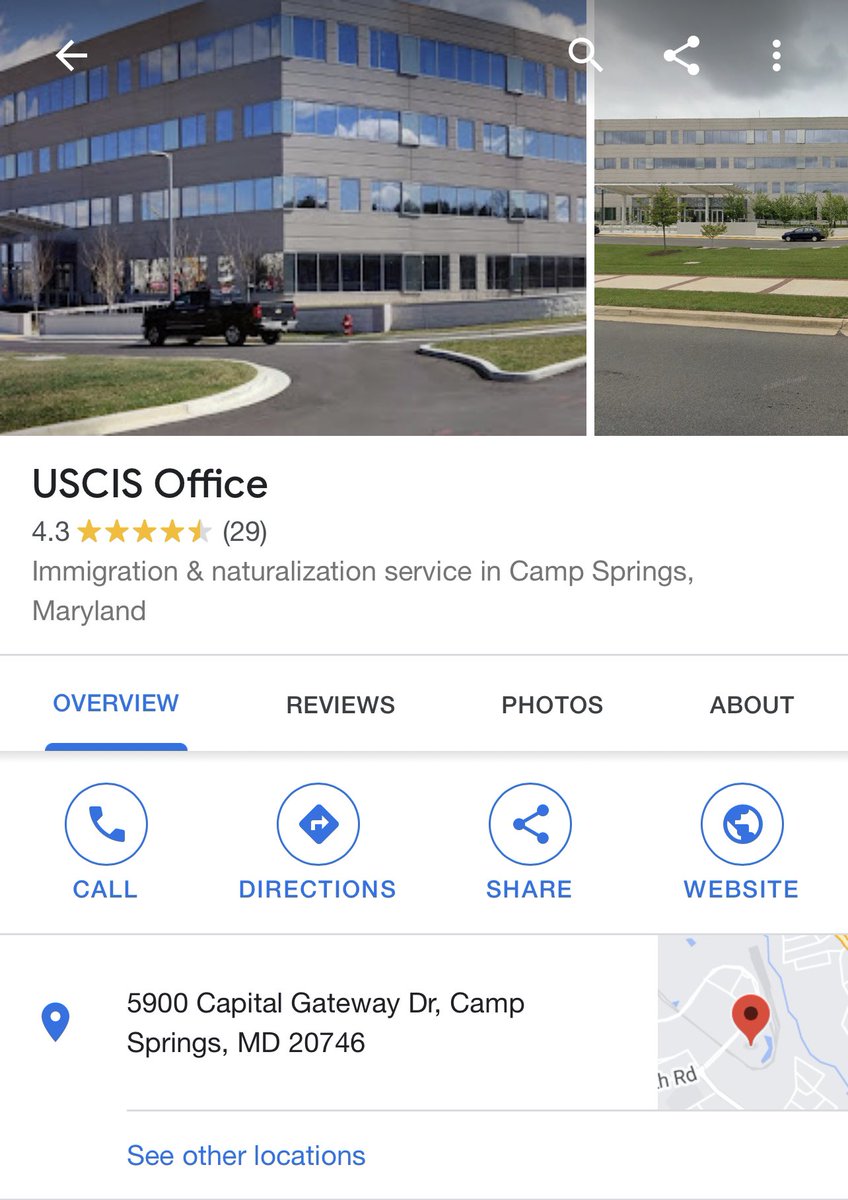This screenshot features a user interface with a clean white background. At the top section, there are two images. The left image is a square-shaped photograph depicting an office building with a road in front, while the right adjacent image is a rectangular shot offering an alternate view of the same building.

Beneath the images, slightly indented, "USCIS Office" is prominently displayed in large black letters. Below the title, there's a star rating of 4.3 displayed through gold stars, with the number of reviews, 29, indicated in parentheses. The subsequent line provides additional details, reading "Immigration and Naturalization Services in Camp Springs, Maryland." 

A light gray horizontal line separates this section from the menu underneath. The menu options include "Overview" highlighted in blue and underlined, followed by "REVIEWS," "PHOTOS," and "ABOUT," all written in uppercase black text. 

Another light gray horizontal line separates the menu from the action icons below. These icons are all blue and listed as follows: "Call," "Directions," "Share," and "Website." Following this is another light gray line, below which lies the location information.

To the left, a location icon is displayed beside the address, "Camp Springs, MD 20746." Adjacent to this is a square Google Map thumbnail featuring a red map pin, providing a visual cue to the location. 

Continuing downward, another light gray line is followed by a clickable blue link stating "See Other Locations."